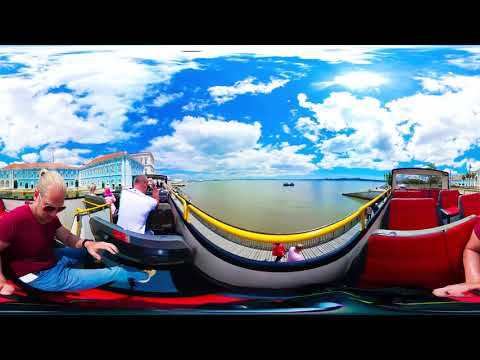In the slightly distorted panoramic photograph, likely taken with a 360-degree effect, we are presented with a tranquil coastal scene viewed from an open-air boat deck. Dominating the left side of the image, a man with blonde hair tied back into a ponytail is seated. He is wearing dark sunglasses, a red shirt with sleeves just below the shoulders, and blue pants. His right hand, adorned with a black wristwatch, is raised, possibly engaging with an electronic device. The boat's seating arrangement has rows with red cushioning, with the seats on the right side facing the camera and those on the left facing away, suggesting the boat's motion is toward the left.

In the foreground, just below the water level, there's a noticeable yellow barrier, likely a handrail, with a light gray walkway beneath it. A black line runs across the top of the walkway. Two figures are seen walking on this path: a man in front wearing a pink shirt, followed by a lady in red. The body of water, visible beyond the yellow barrier, appears brownish in color. To the far left, a tall building with white walls and a blue side, topped with a red roof, signifies urban architecture along the coastline. Above, the sky is a blend of white and gray clouds with patches of blue, allowing bright sunlight to filter through on the right. Additionally, a small vessel can be seen in the distance, contributing to the serene maritime atmosphere.